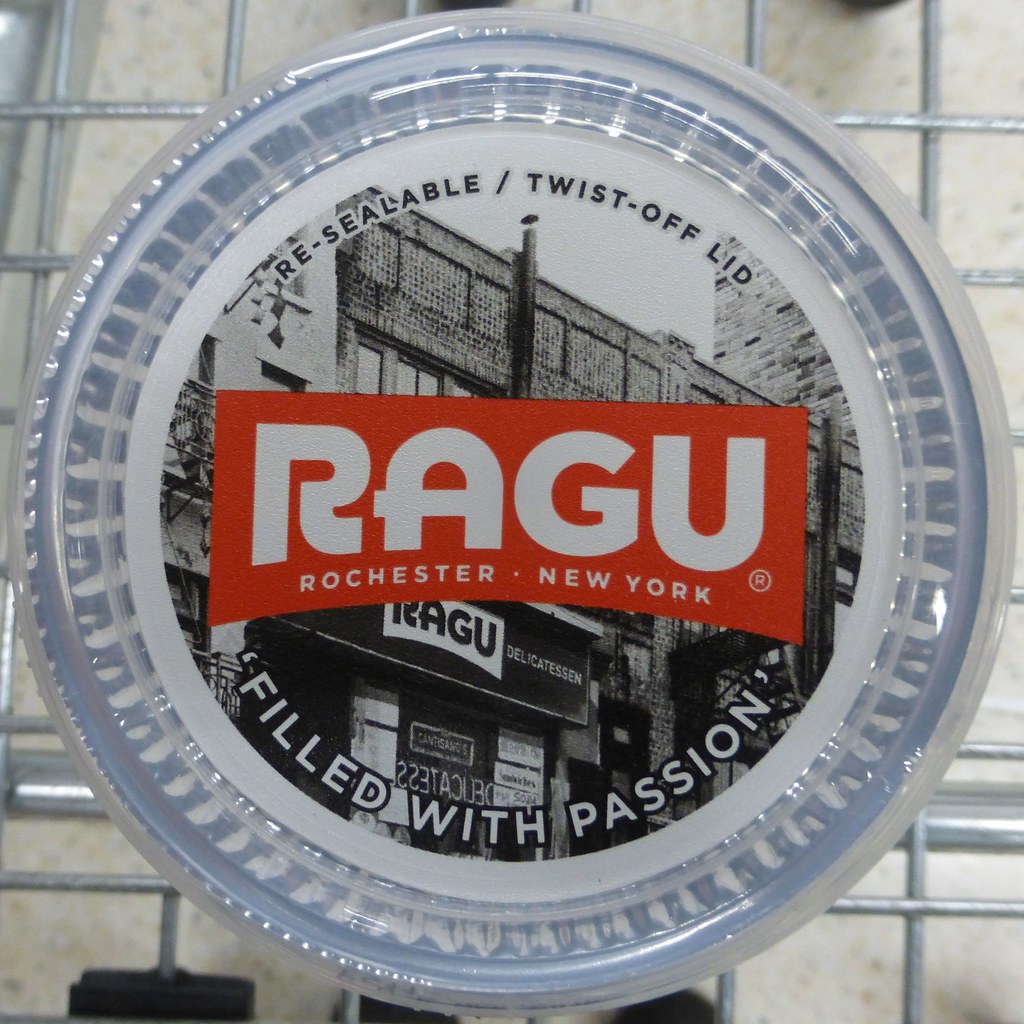The image showcases the top of a Ragu jar, prominently featuring its resealable twist-off lid with a clear plastic cover. The lid itself is circular and designed with a vivid red background displaying "Ragu" in bold, white letters set within a rectangle. This central red bar is flanked by "Rochester, New York" text, indicating its origin. Surrounding the red bar is a monochrome image of a two-story building, the lower part resembling a storefront with the words "Ragu Delicatessen" and the upper part depicting a brick structure. The rim of the lid is light blue, with additional text in black that reads "resealable twist-off lid" at the top, and white lettering with a black outline that says "filled with passion" at the bottom. The jar appears to be placed inside a grocery cart, evident from the metal wiring visible around it, suggesting the photo was taken in a shopping environment.